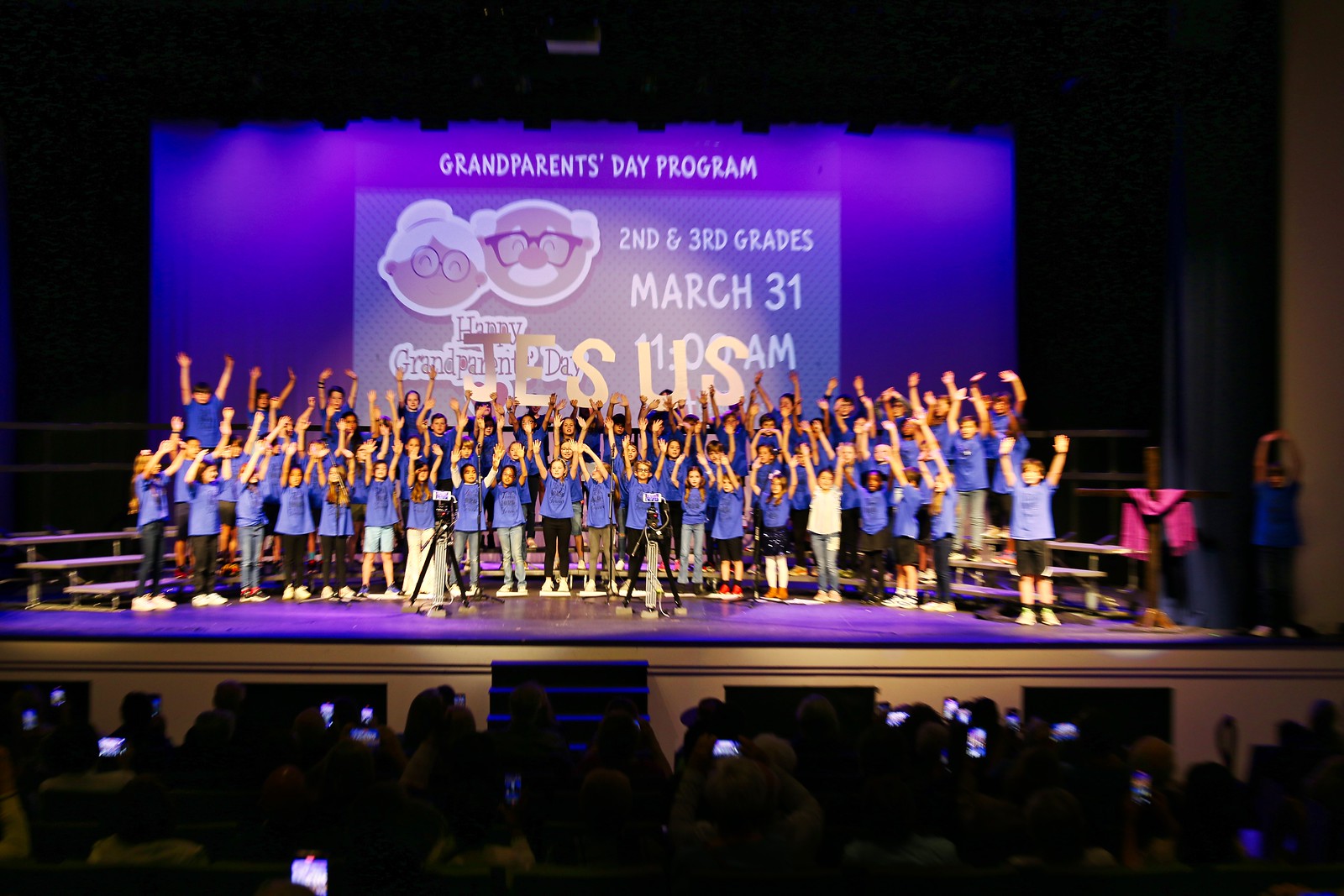This full-color photograph captures an indoor school event, the Grandparents Day Program for second and third grades, held on March 31st at 10 a.m. The scene is set on a stage with a backdrop featuring a large screen displaying white text and cartoon images of a grandma and grandpa. At the top of the screen, a banner reads: "Grandparents Day Program, second and third grades, March 31st." On the stage, a group of children, mostly wearing blue shirts with one child in white, are standing on risers. They all have their arms up in the air in what appears to be a coordinated gesture. To the far right of the stage, a cross draped with a pink shawl is visible. The audience at the bottom of the photograph is engaged, many with their phones up, presumably recording the performance. Additionally, a couple of cameras on the stage are also capturing the event. The setting suggests a hall or theater, enhanced by black curtains and a blue-themed background.